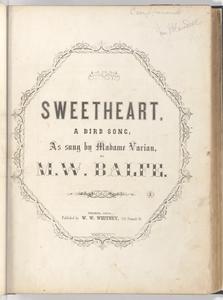The image is a photograph of what appears to be the title page of an antique book, likely from the 1800s. The book's aged, cream-colored paper features a prominent title in large, brown text that reads "Sweetheart." Beneath the title, in smaller text, is the subtitle "a bird song." Below this, in an old English font, it says "As Seen by Mahams Varissa." The author's name, "M. W. Balfe," appears in larger, more straightforward text, "M.W." followed by "M. W. B-A-L-F-E." This text is framed by an ornate octagon-shaped border. The paper also shows signs of age, with a yellowed appearance and possibly a handwritten pencil inscription or owner's name in the upper right corner. The overall texture of the cover has a slightly 3D, tactile quality, indicating it might be a booklet or a transcription of a song, resembling a sheet of music. The book conveys an antique aesthetic with its classic and somewhat worn look.